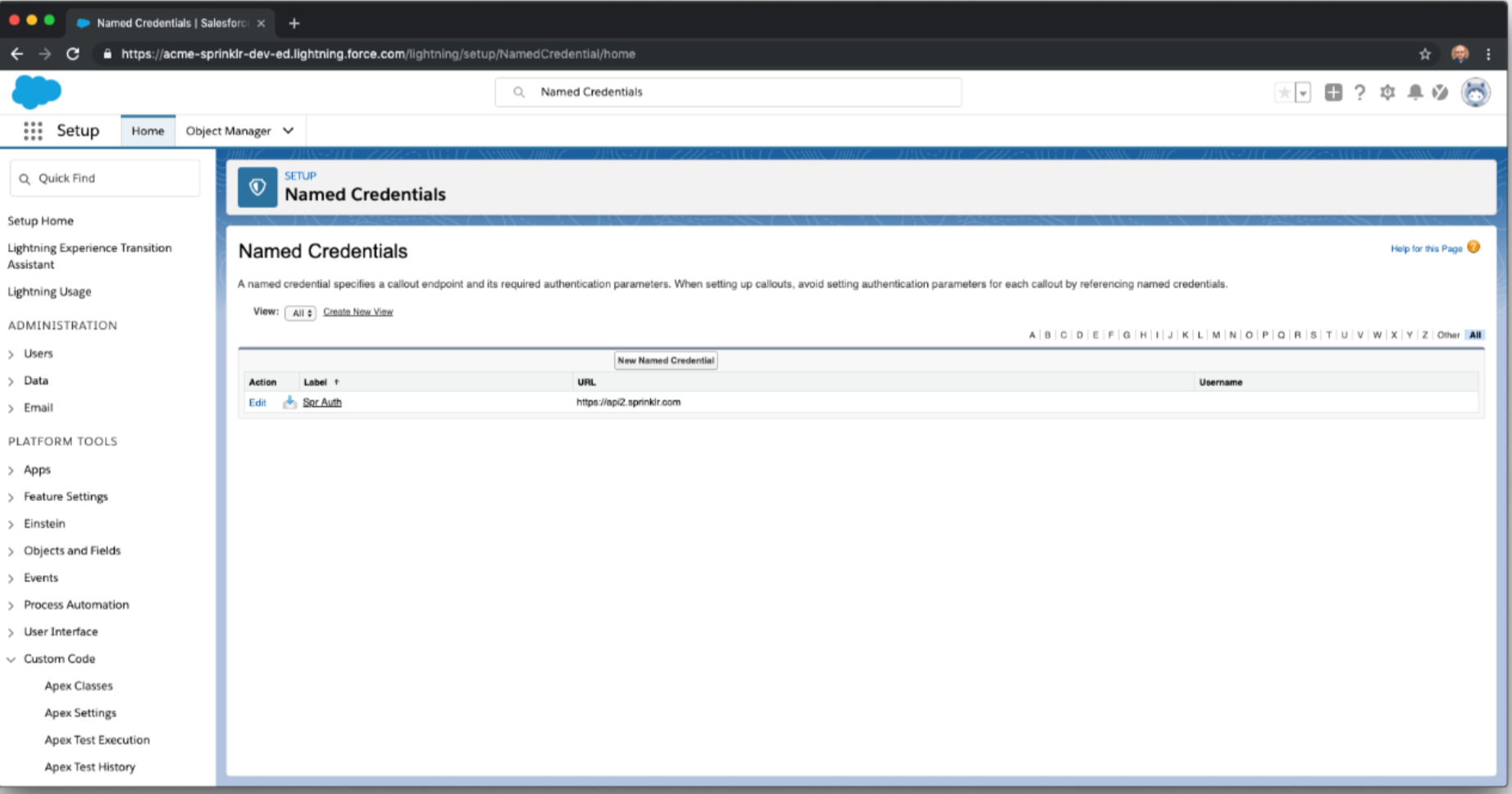The image depicts a screenshot of a web browser window on a Mac-based system. At the top of the window, there is a black bar running across, with three iconic circles—red, yellow, and green—situated in the upper left corner, indicating the typical control buttons for closing, minimizing, and maximizing the window. Below this, a single tab is open, featuring a cloud icon at the top, suggesting some sort of cloud-based application or service.

The main background of the page is white. Beneath the cloud icon, there are several tabs labeled "Setup," "Home," and "Object Manager," arranged horizontally in the upper left section of the interface. Below these tabs, on the left side, is a "Quick Find" search bar, followed by various sections labeled "Administration" and "Platform Tools." Each section includes a list of options for further navigation.

On the right side of the page, there is a section titled "Named Credentials." Under this heading is a text box where users can presumably enter information, and a file is also visible within this area, indicating that file management or uploading features might be available.

Overall, the image shows a detailed administrative interface likely belonging to a cloud-based platform, with clear sections for easy navigation and management tasks.